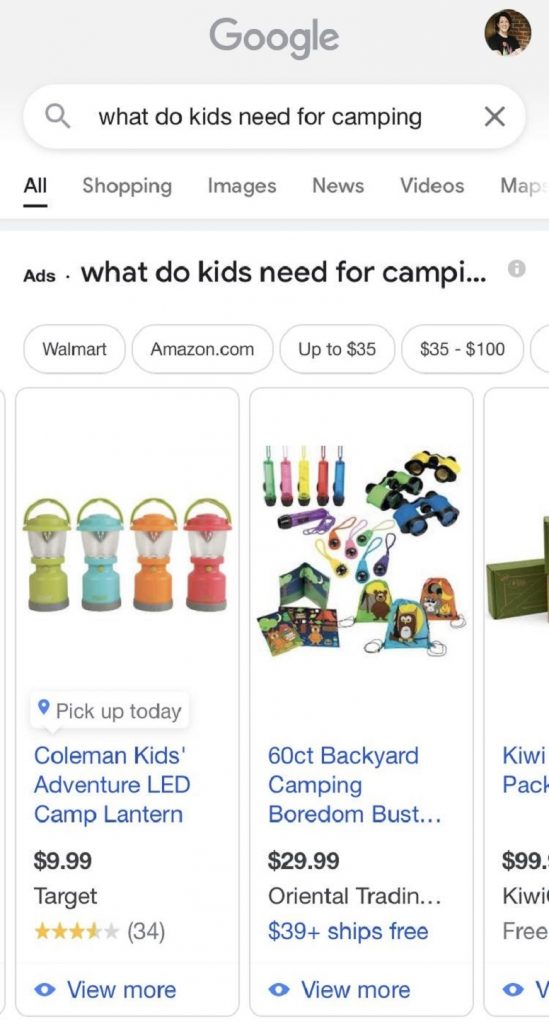The image displays a Google search results page with a gray navigation bar at the top bearing the Google name in a monochromatic gray color instead of the usual multi-colored logo. The search query entered is "what do kids need for camping" and the results show under the "All" tab, with other available categories including "Shopping," "Images," "News," "Videos," and "Maps."

Among the search results, there are ads featuring products from retailers like Walmart and Amazon, displaying a pricing range from $35 to $100. One prominent ad shows a color image of "Kohl's Kids Adventure LED Camp Lanterns" available in green, blue, orange, and red. The lanterns are priced at $9.89 each and are sold at Target, holding a 4 out of 5-star rating based on 34 reviews. Below the ad, there's a clickable "View more" link in blue.

Another suggestion in the search results is a 60-count "Backyard Camping Boredom Bust," available from Oriental Trading, priced at $29.89 and $39 with free shipping. This item also has a "View more" option.

Finally, there's partially visible information about a product referred to as "Kiwi something pack," priced at no less than $99, though the full description is cut off.